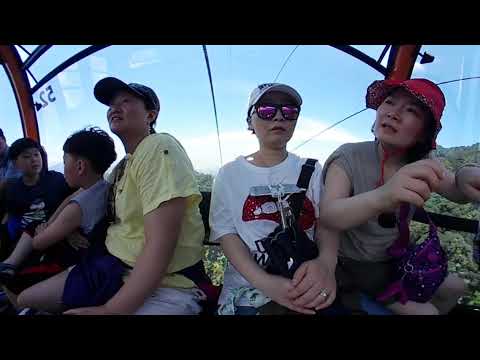In this vibrant daytime scene, a group of six people are captured inside a glass-enclosed skylift, suspended above a lush forest with treetops stretching below and a blue sky dotted with clouds above. The group includes three women, two boys, and one more person partially obscured. On the far right, two women seem closely acquainted; one wears a red bucket hat, a tan shirt, and has a purple fanny pack in her lap, while the other sports a white hat, sunglasses, and a red and white shirt, accessorized with a black shoulder bag. To their left, another woman wears a light yellow t-shirt and a black baseball cap, tenderly wrapping her arm around a young boy in a gray t-shirt. Another child, slightly in the background, is dressed in a black t-shirt. The cosy setup inside the skylift offers clear panoramic windows that frame the scenic and serene landscape outside.